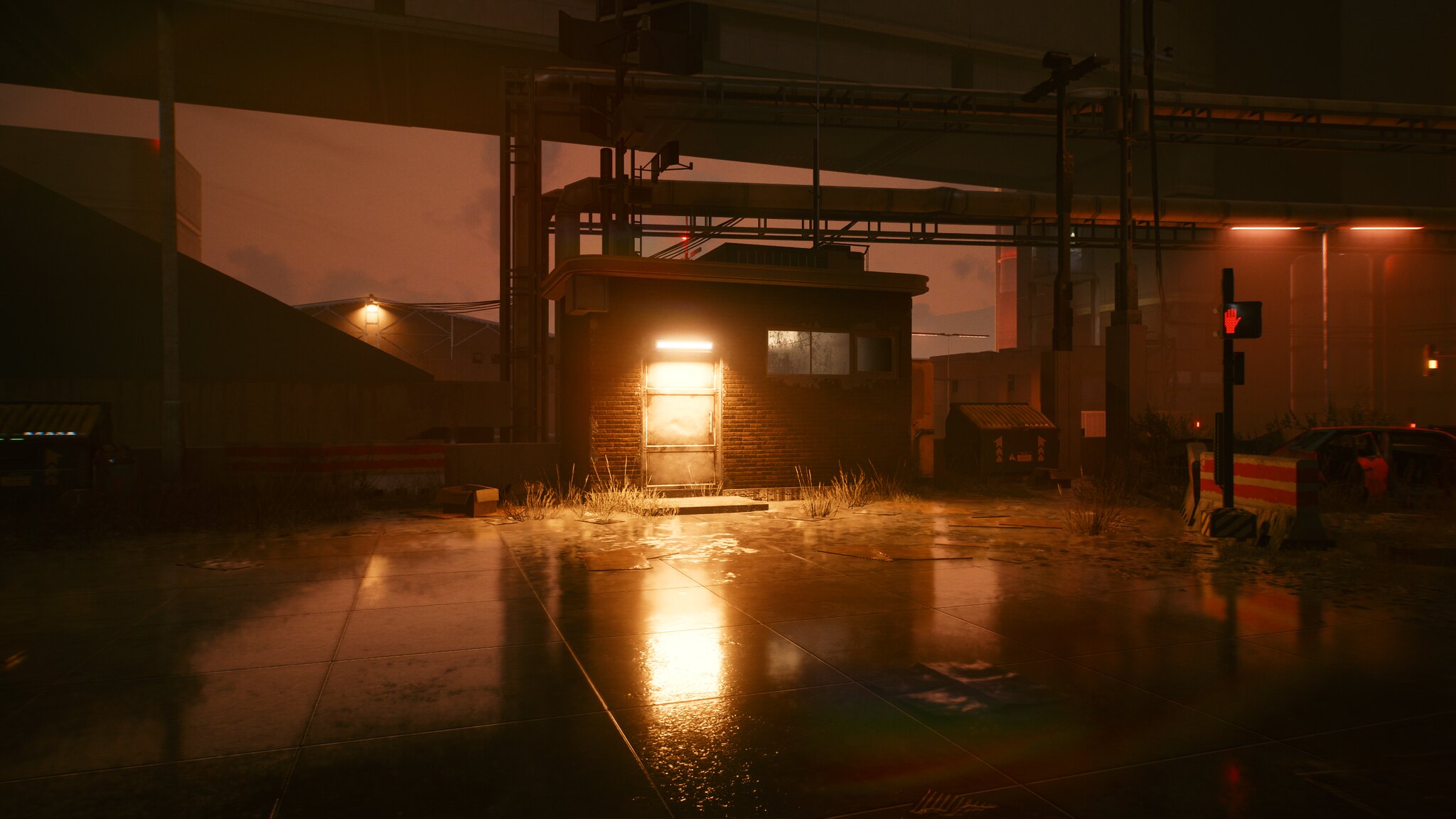A wet, reflective tiled ground stretches into the distance, creating a mirror-like effect. Towards the horizon, a patch of dry grass is visible, juxtaposing the gleaming tiles. In the right mid-ground stands a sign on a pole that reads "STOP" with an illustration of a hand, providing a stark command in the scene. On the far left, a building with a white door and a lit window glows warmly against the backdrop of the overcast, gray sky filled with scattered clouds. Above the building, there is an elevated highway. The foreground contains various objects that add depth to the scene, contributing to an overall atmosphere of stillness and subtle complexity.